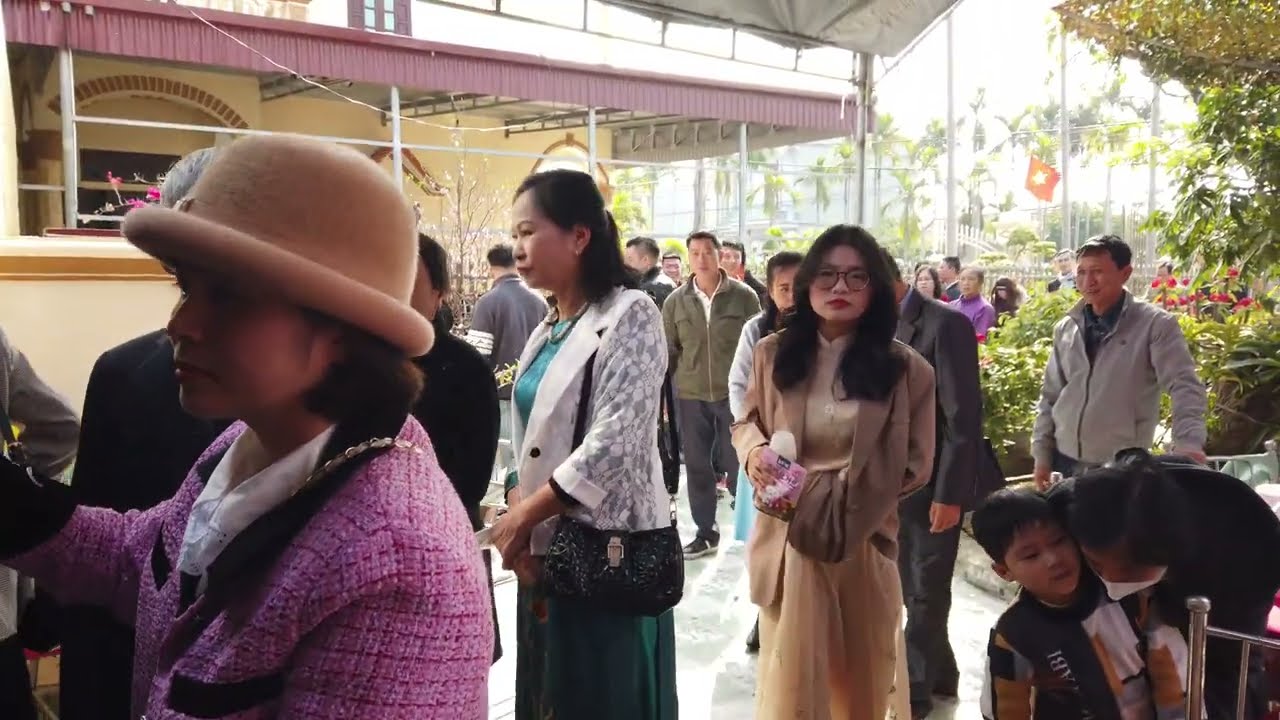The photograph captures a bustling crowd gathered in an open-air area, possibly in Vietnam, suggested by the presence of a Vietnamese flag in the background. The diverse group is moving or looking towards an unseen destination to the left of the image. On the far left, a woman in a pink coat and a brown bowler hat gazes to the left, with an Asian woman in a green dress and white coat slightly behind her, holding a black purse. To the right of the woman in green, another Asian woman with longer black hair, glasses, red lipstick, a light brown dress, and a brown coat holds a pink item in her hand. Further back, an Asian man in a gray sweater is visible. In the bottom right corner, a small child interacts with someone leaning over from behind. The crowd blends into the background, where a yellow building with reddish-purplish doorways and a purplish roof stands on the left. Additional details include a tan building with steel supports and a large cloth-like ceiling behind the crowd. The distant background hints at green foliage, pink flowers, and tall trees, partially obscured by the bright sky. Some people wear casual attire like sweatpants, but many are in warm, outdoor clothing.